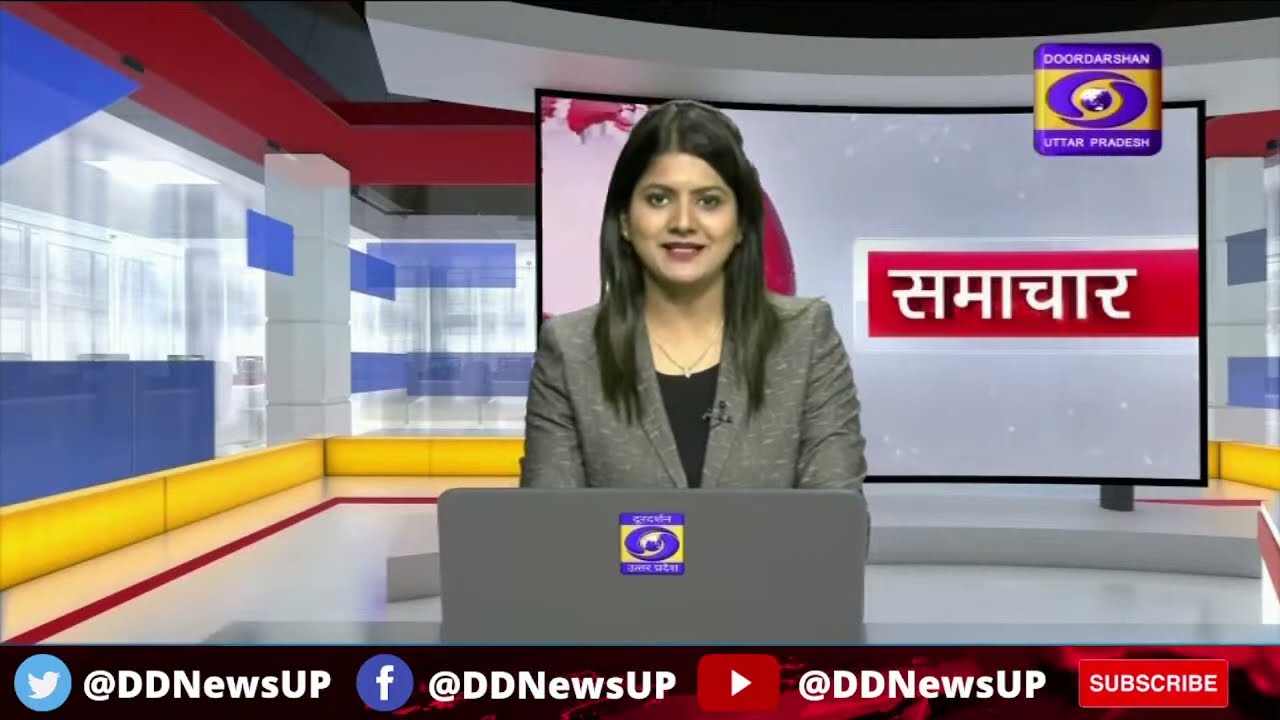The image is a detailed screenshot of an online news broadcast featuring a female presenter dressed in a gray blazer and black blouse, accessorized with a necklace. She stands in a digitally rendered environment resembling a futuristic office room, accentuated with a flat-screen TV behind her that displays presumably foreign or possibly Arabic text. In front of her is an open laptop, indicating her engagement with digital content. The woman, who has long brown hair, is centered prominently within the frame. The visual composition includes social media callouts at the bottom edge of the image, listing Twitter, Facebook, and YouTube icons in order from left to right, with the handle "DDNEWSUP." A red rectangular strip with the word "Subscribe" in white reinforces the call to action. In the upper right-hand corner, a yellow rectangular logo featuring a circular disc with a planet hints at the news company's identity. The setup suggests a green screen was utilized to create this sophisticated virtual studio.